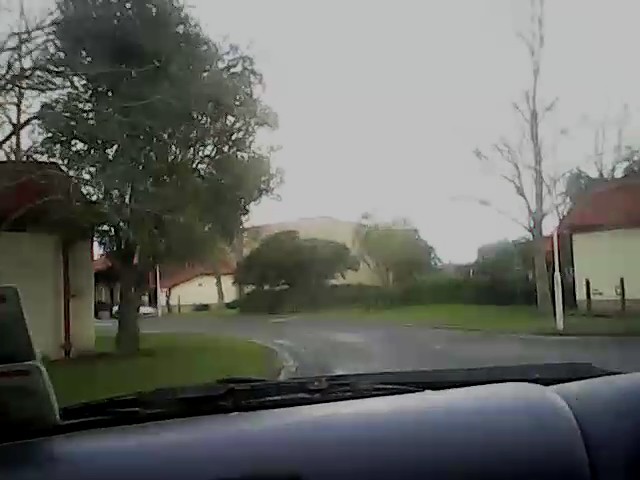A photograph captures a scene seemingly from inside a vehicle, possibly taken by a driver, passenger, or a dash cam. The image showcases a quaint residential area featuring a narrow, dark asphalt-paved street. Flanking the road are several houses or buildings, all adorned with light-colored siding and brown roofs, hinting at a uniform architectural style. On either side of the street, patches of grass and sporadic trees dot the landscape, adding a touch of greenery. The sky overhead is pale gray, indicating a cloudy, overcast day, setting a serene, subdued atmosphere. The shot encompasses the essence of a calm suburban neighborhood, void of any text or superimposed elements.